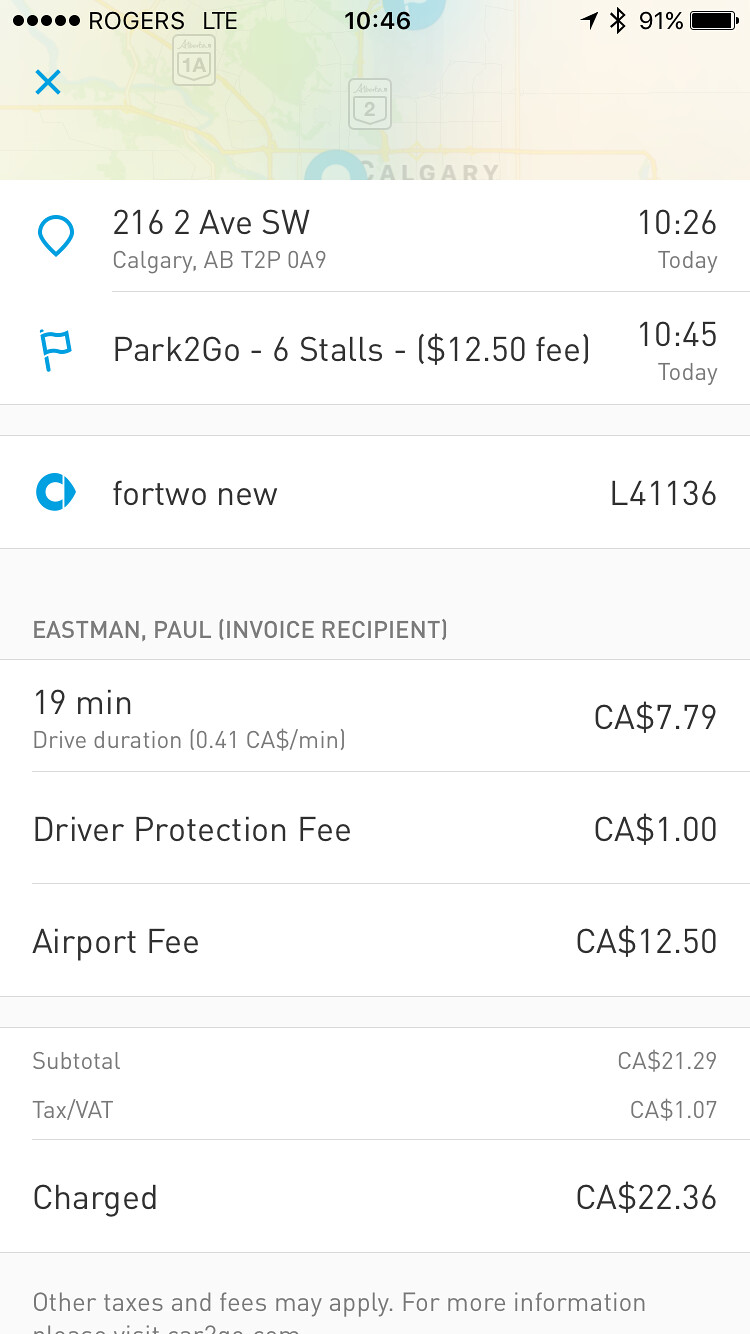The image is a color screenshot taken from a phone in portrait orientation. It shows various details with a focus on charges incurred during the day, including parking and airport fees. At the top left corner, there are five black signal circles next to "Rogers LTE." The time at the top center is 10:46, and the right side shows an arrow symbol, a Bluetooth symbol, and a battery icon at 91%. Below this, there is a faint, blurred map of Calgary. 

Under the map is a location pin indicating "2162 AV SW" and the address "Calgary, AB T2P 0A9". The time on the right reads "10:26 today." The next section highlights a blue flag icon with text next to it that states "Park to Go, 6 stalls, $12.50 fee" at "10:45 today."

Further down, it displays "42 new" and "L41136," followed by "Eastman Paul (invoice recipient)" and details of a "19 minutes drive duration" costing "CA $7.79." 

Additional charges include a "driver protection fee" of "CA $1.00" and an "airport fee" of "CA $12.50." The subtotal is listed as "CA $21.29," with "tax/VAT" at "CA $1.07." The total amount charged is "CA $22.36." The image notes that "other taxes and fees may apply," though the bottom is cut off, leaving the rest unseen.